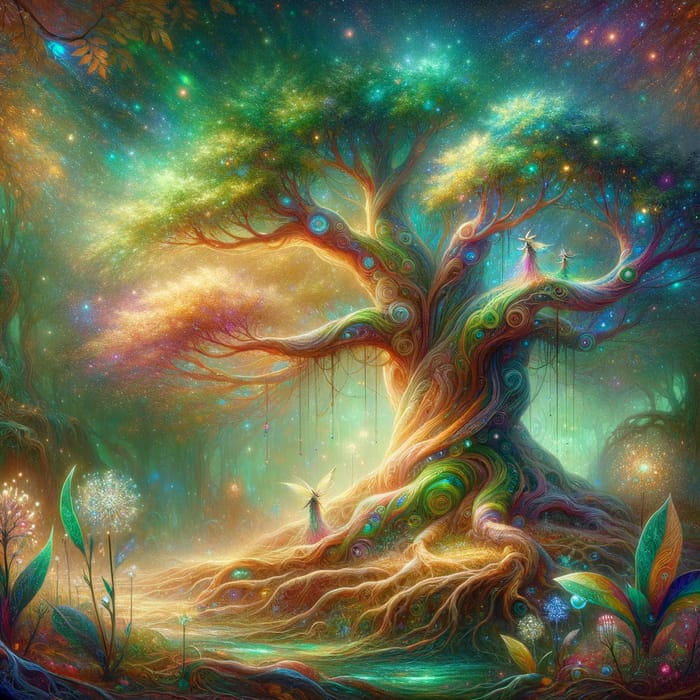This is a mesmerizing digitally created or hand-drawn fantasy art piece depicting an enchanted forest. At the center of the image stands a grand, multicolored tree with squiggly, captivating patterns and curlicue designs. The tree's trunk and branches exhibit vibrant hues of greens, oranges, yellows, and rainbow swirls, adding to the magical aura. The foliage is predominantly green but includes a golden-hued branch on the left side. To the left foreground, there are delicate dandelions, while to the right, ferns and small flowers are visible, enhancing the lushness of the forest. The background, although somewhat foggy, reveals an intricate woodland with branches intertwined. Amidst this mystical scene roam fairies, adding to the whimsical charm. Two fairies with witch-like hats—one pink, one green—perch on a lower branch, while another fairy dressed in a pink and green dress stands near the base of the tree. Additionally, there's a suggestion of a river flowing beneath the roots, with fairy lights and sparkling fairy dust twinkling throughout the image, completing this enchanting masterpiece.